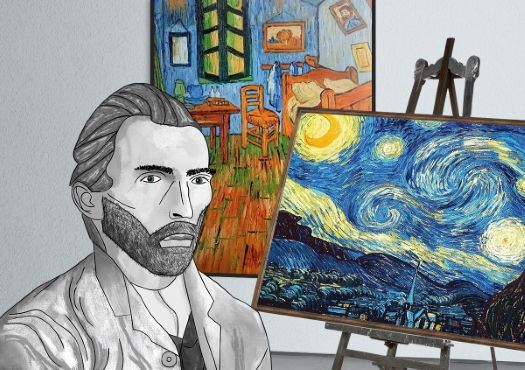The image features a detailed pencil drawing of Vincent van Gogh in black-and-white, portrayed from the torso up. Van Gogh is depicted with a combed-back hairstyle, a beard, thick black eyebrows, and is dressed in a light-colored coat paired with a dark waistcoat. Notably, he has both ears intact. Behind him, the background showcases two of his famous paintings in vivid color. On the right, placed on an iron easel, is the iconic "Starry Night," which illustrates a swirling night sky in blue and yellow above a village. To the left, pinned against a white wall, is the painting "Bedroom in Arles," characterized by its stylized depiction of a room featuring a brown chair, a wooden bed frame, clothes hanging on the wall, windows, colorful bottles, and a nightstand, all against a blue wall. The contrast between the monochromatic sketch of van Gogh and the vibrant hues of the paintings highlights the artist's dual existence in art and life.